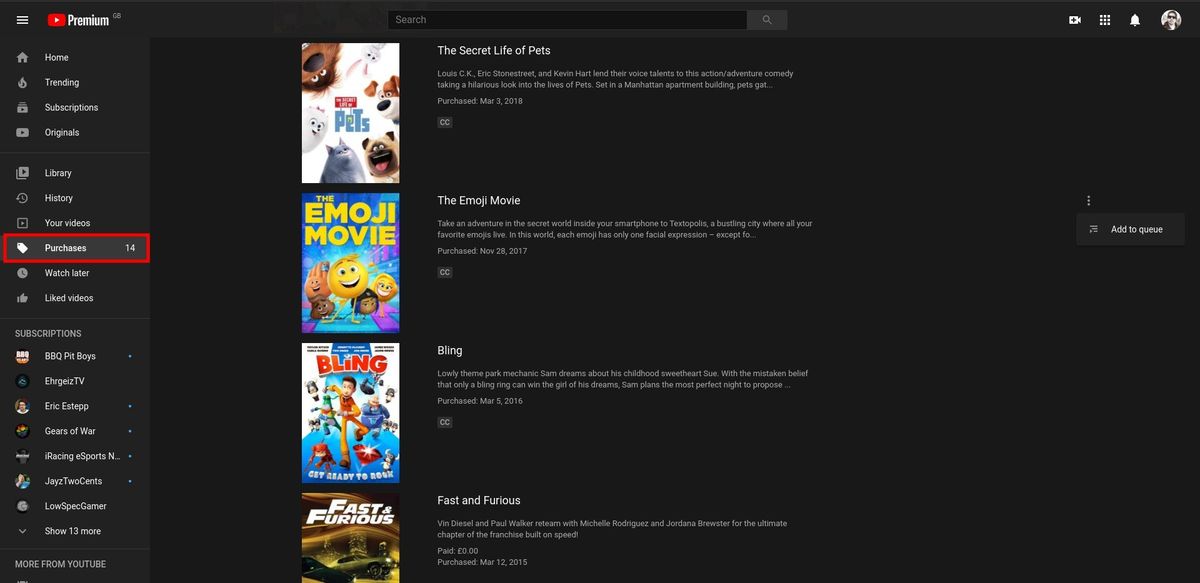This is a detailed screenshot of YouTube Premium's home page, where the primary background is black. In the top left corner, three horizontal white lines, stacked one above the other, denote a menu icon. To the right of this, the well-known YouTube play button, colored in red, is present. Adjacent to this, the word 'Premium' is displayed boldly in white font.

Centrally positioned on the page is an elongated search bar, with the placeholder text "Search" inside it. To its right, a small square containing a magnifying glass icon protrudes from the bar to signify the search function. Moving rightward, there are several icons: a profile picture, a notifications bell, three vertical dots indicating additional options, and a camera icon.

On the left side, under the premium header, there are four primary icons: 'Home,' 'Trending,' 'Subscriptions,' and 'Originals.' Directly below these, additional categories are listed: 'Library,' 'History,' 'Your Videos,' and 'Purchases'; the 'Purchases' category is highlighted with a red rectangle, accompanied by the number 14.

Further down, there's an option for 'Watch Later' videos, followed by a list of eight clickable subscription channels. Below this list, a link labeled 'Show 13 more' is present. At the very bottom of the sidebar, a section titled 'More from YouTube' appears.

Just under the search bar, shifting a bit to the left, you notice a cover line-up for four movies, with their lower edges slightly cropped. To the right of each cover image, the movie's title is written, followed by two lines of additional information and the purchase date. The movies listed include "Patched," "The Emoji Movie," "Bling," and "Fast and Furious." Near the right edge of the page, a gray tab labeled 'Add to queue' in white text is positioned next to "The Emoji Movie."